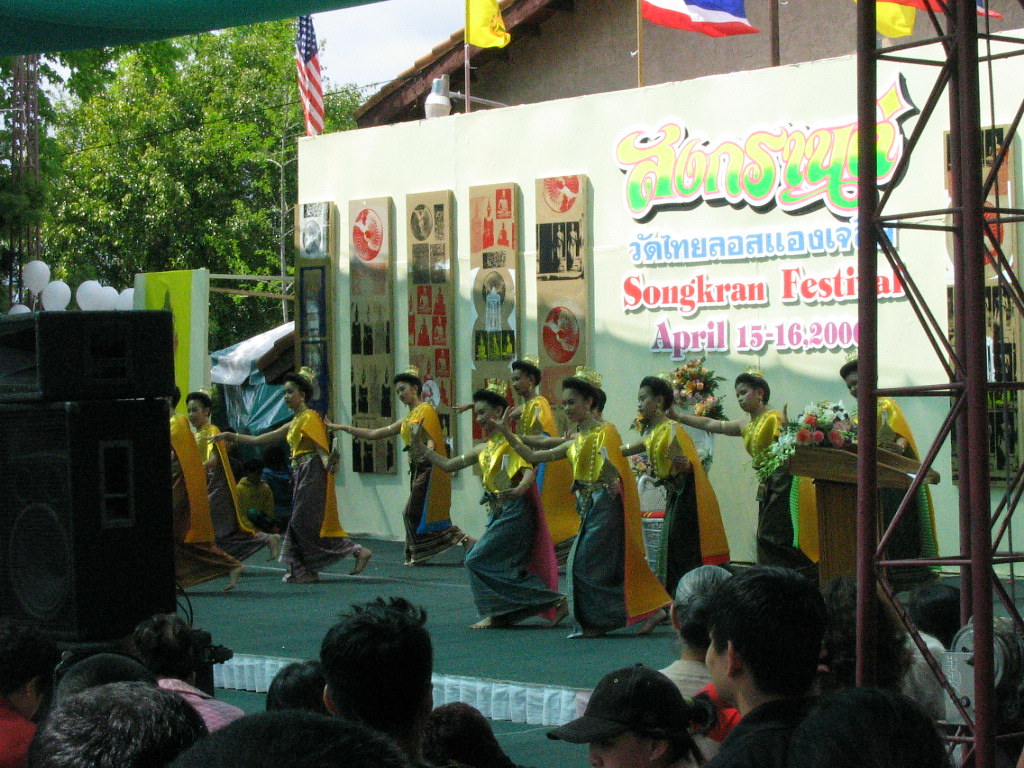This photograph captures an outdoor scene at the Songkran Festival held from April 15th to 16th, 2000. Featured prominently are nine women dressed in vibrant yellow and gray costumes, consisting of yellow tops and capes paired with gray skirts. They are adorned with yellow-gold necklaces and crowns, and they are either barefoot or wearing sandals. The performers are positioned centrally on a short, raised stage, pointing towards the left. 

Behind them is an ornate backdrop with inscriptions in multiple colors, including the prominent “Songkran Festival, April 15th-16th, 2000.” The backdrop also consists of other designs and text in various stylings. Flags are suspended above the stage, including an American flag, a yellow flag, and a red, white, and blue flag. Additionally, white balloons add to the festive atmosphere.

In the foreground, an audience observes the performance, their heads visible just above the stage. On the left side of the image, a large black speaker is noticeable, suggesting the presence of audio equipment. The composition and festive elements imply the celebration might be taking place in the United States, despite being a Thai festival.